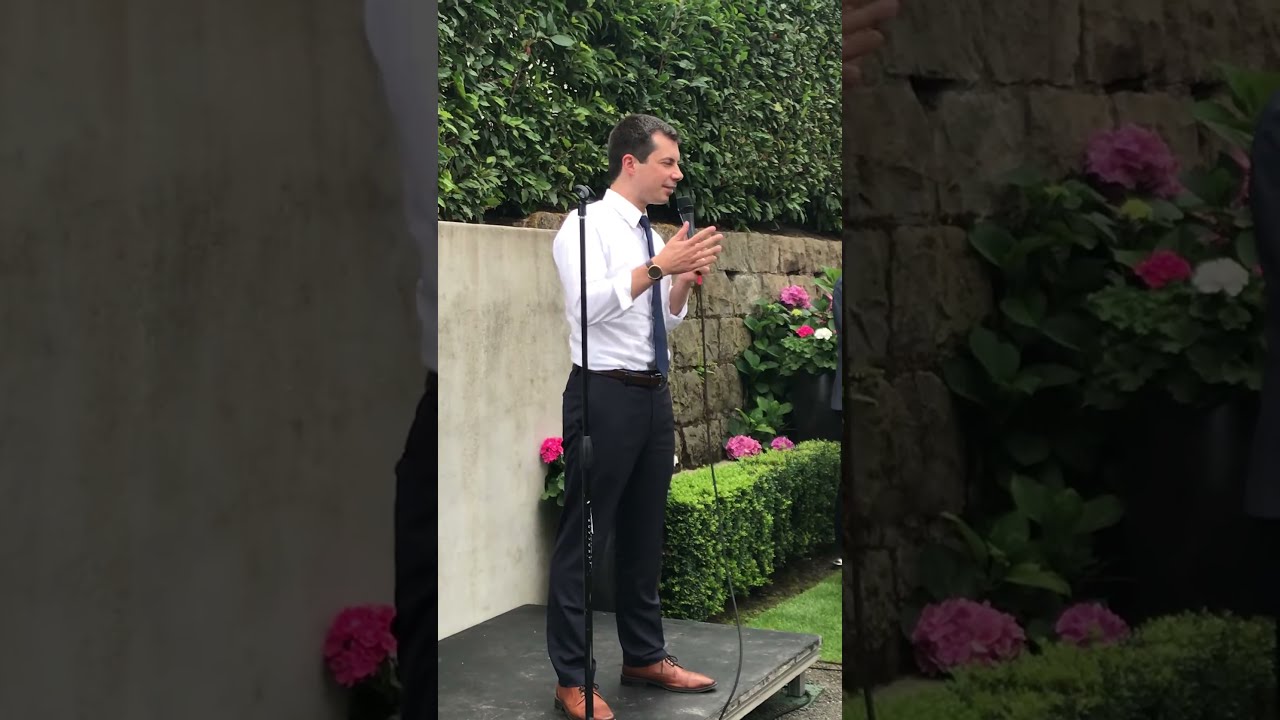In this outdoor photograph taken in a yard, a young white man in his 30s stands confidently on a small black stage, holding a microphone in his left hand as he addresses an unseen audience. He is attired in a white shirt, a dark tie, black slacks, and brown shoes, with a black wristwatch adorning his right wrist. His short, dark hair is neatly styled, and he has a calm, composed expression. To the right of the stage, a small hedge is adorned with vibrant purple, pink, and white flowers, adding a touch of color to the scene. Behind him, a combination of a stone wall and a concrete wall serves as a backdrop, extending upwards with lush green bushes. The image is thoughtfully composed, capturing the man mid-speech in a serene garden setting.